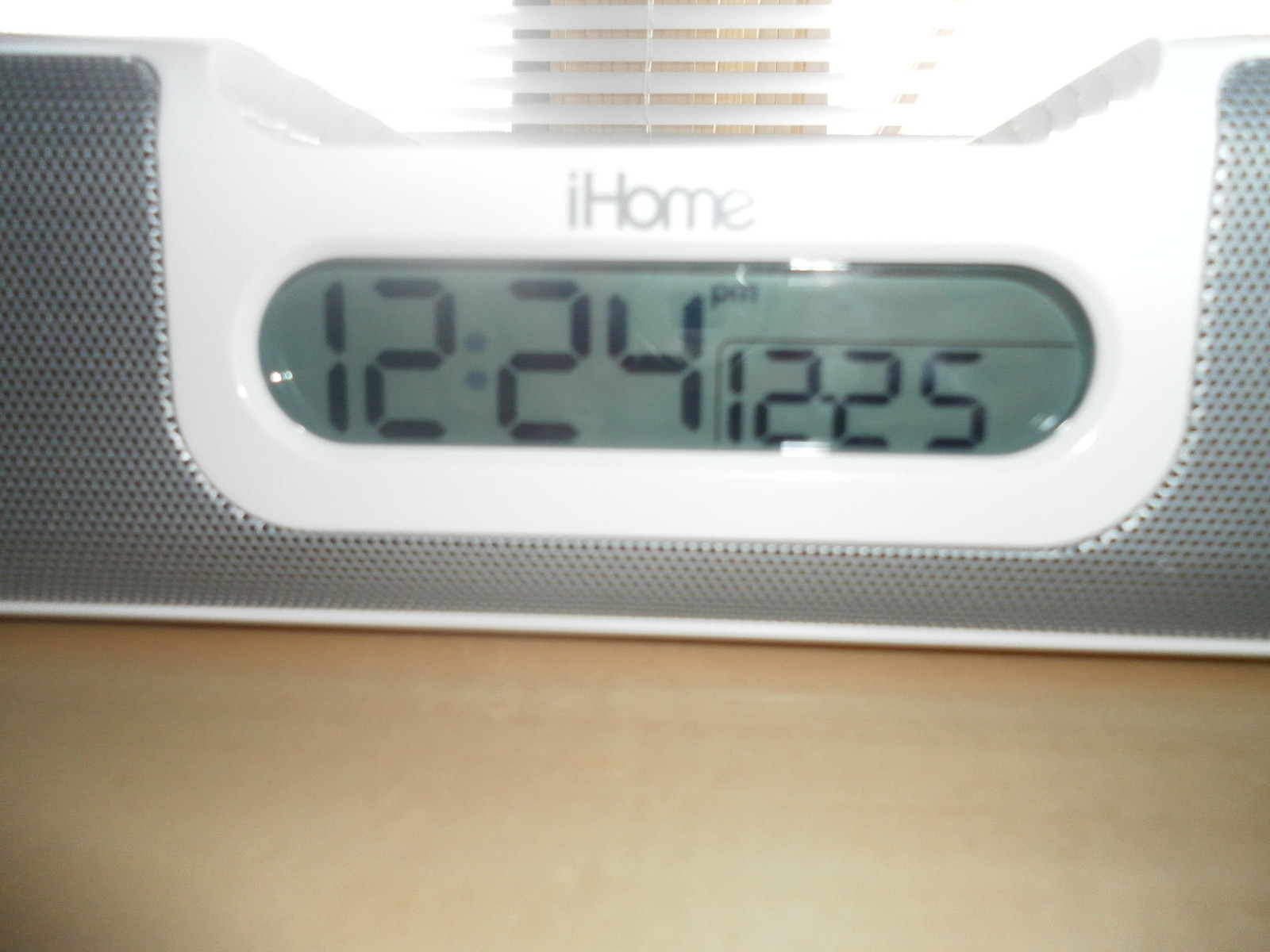The image is a close-up of an iHome alarm clock, prominently displaying its sleek and modern design. The alarm clock features a raised, vent-like structure at the center top, characterized by a metal mesh with very small holes in the cover. The metal cover surrounding the digital display is a plain white, contrasting with the light grey iHome logo positioned just below the vent. The digital display, resembling a horizontal capsule, shows the time as 12:24 p.m. with a small box on the lower right side indicating 12.25, possibly signifying the date Christmas Day. The alarm clock is mounted on or positioned against a tan-colored wall. This is a close-up shot likely taken in a bedroom, with open linoleum lines discernible in the background, contributing to the bright and light atmosphere of the scene. The photograph focuses solely on the alarm clock, with no people or additional text in view.